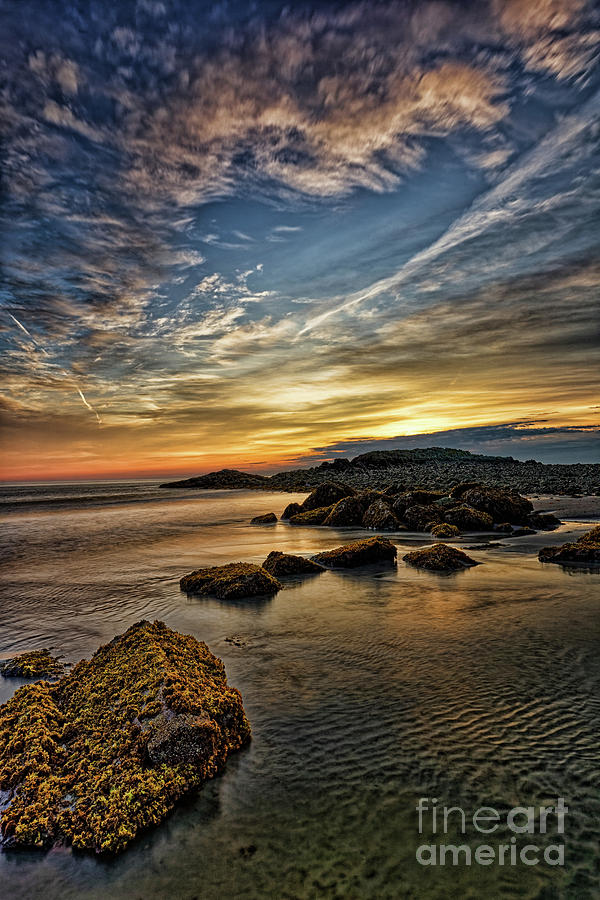The image captures a serene sunset over a body of water with various rock formations protruding in the foreground and background. The horizon showcases a vibrant sunset with the sky transitioning from bright gold, yellow, and white near the horizon to a darker blue shade adorned with streaks of light brown and white clouds at the top. The clouds closer to the horizon are illuminated with shades of brown, yellow, and vibrant orange, framing a bright, light yellow spot where the sun is setting.

In the foreground, on the bottom left-hand side, there's a rock covered in yellow and green algae or seaweed. On the right side of the image, a cluster of four rocks juts out of the water, and behind them, a mound of boulders is piled together. Further into the background on the right, a spit of land extends out into the water. You can see the waves rolling in, clearly defining the surf line where they meet the beach. The sandy beach shows signs of erosion from the constant ebb and flow of the waves.

In the bottom right corner of the picture, the words "Fine Art America" are written in gray text.